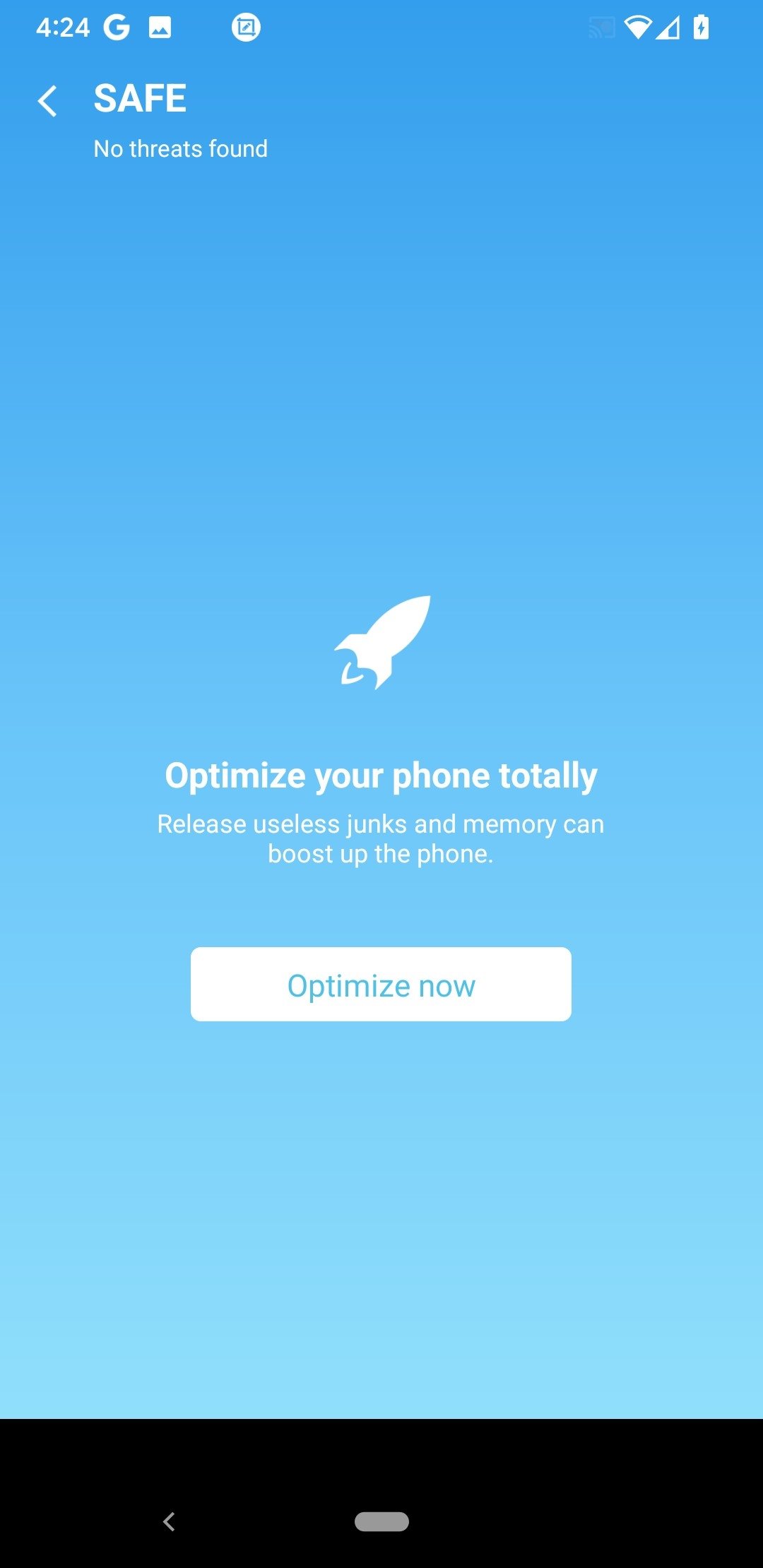The image features a blue gradient background that transitions from light blue at the bottom to dark blue at the top. Central to the design are several key icons: "424," a "G," a battery symbol with a lightning bolt indicating charging status, and a safe with a backward arrow signifying no detected threats. Additionally, the image includes depictions of a spaceship and a rocket ship, emphasizing a theme of optimization and efficiency.

At the bottom, a white rectangular button prominently displays the text, "Optimize Now." The image suggests that optimizing your phone can eliminate useless junk and free up memory, thus enhancing the phone's performance. Finally, a black footer contains a gray left arrow on the left side and an "R" in the middle.